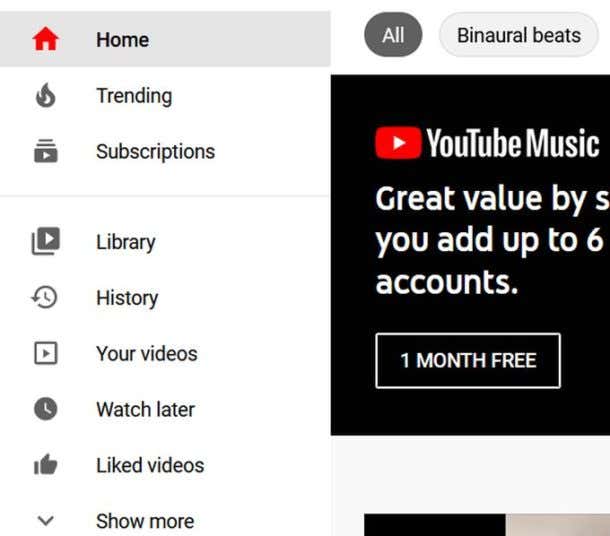The image displays a YouTube interface set against a white background. On the left side, there is a vertical navigation bar that is left-justified with a list of options. The top option labeled "Home" features a red home icon, while the text beneath it is gray. The subsequent navigation options are white and include "Trending," "Subscriptions," followed by a gray dividing line, and then "Library," "History," "Your Videos," "Watch Later," "Liked Videos," and "Show More."

On the right side of the image, there are two button options labeled "All" and "Binaural Beats." The "All" button is dark gray, whereas the "Binaural Beats" button is light gray. Below these buttons, there appears to be a partially visible black banner, showing only a section with the YouTube logo (a red rectangle with a white play button) alongside the text "YouTube Music."

Further down, the banner contains promotional text that reads: "Great value by S You add up to six accounts." Below this text, there is a black button with white text offering a "One Month Free" trial.

Additionally, there is a bar beneath these elements that is black on the left and transitions to white or gray on the right, indicating that the image is partially cut off on the right edge. The overall color scheme of the image includes black, white, red, and gray, contributing to a clean and modern aesthetic typical of YouTube's interface.